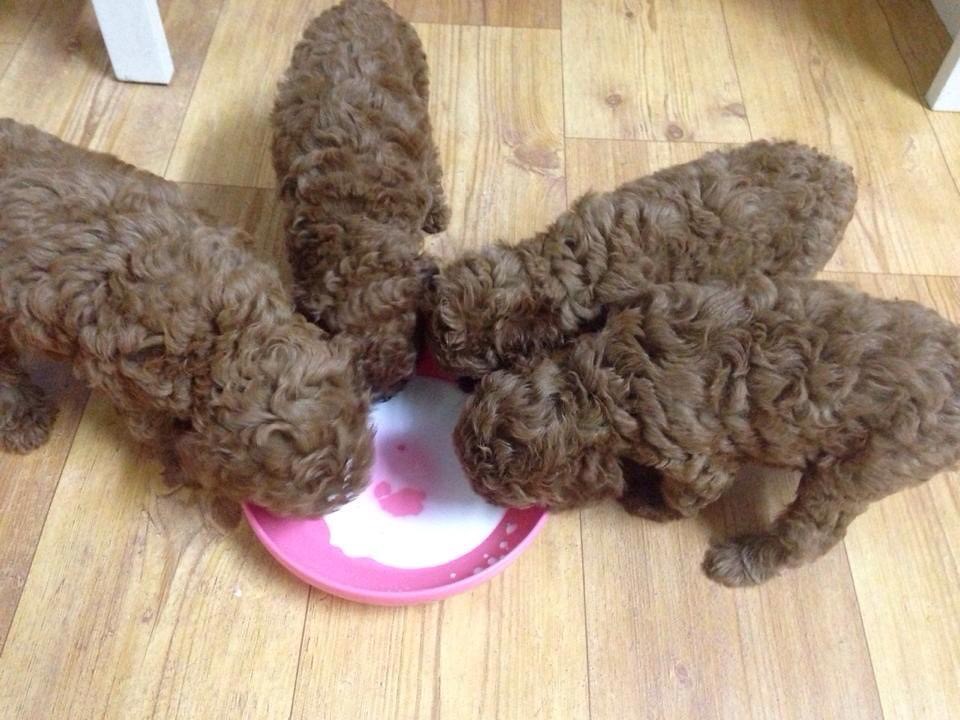This photograph captures an adorable scene of four small, cocoa brown poodle puppies with very curly fur, drinking milk from a shallow pink bowl. The image is taken from an overhead perspective, showing the puppies huddled closely together in a semi-circle around the bowl, their attention entirely focused on drinking. The pink bowl, which has a resemblance to an upside-down frisbee or a prism, sits on a lightly scratched pine wood plank floor. Flecks of sunlight highlight parts of the scene, drawing attention to the puppies' fluffy fur. In the background, there are two white legs of a piece of furniture, possibly a table or stool, positioned at the top left and top right of the frame. The milk in the bowl is nearly gone, with only a little left in the center, reflecting the puppies' enthusiasm.